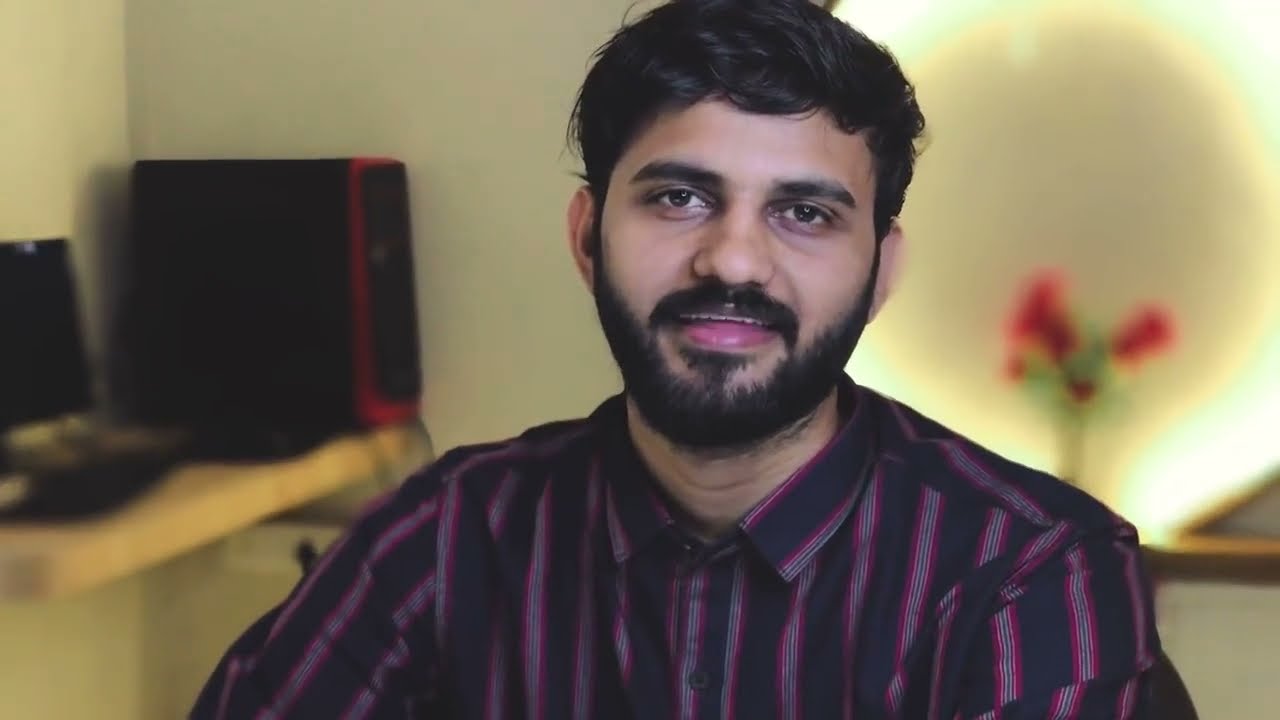In this photograph, a man of possibly Indian or Middle Eastern descent is depicted chest-up, seated in an office environment with a blurred background. The man, who has dark hair styled to the side and a dark, full beard with a goatee, is wearing a dark blue button-down shirt featuring vertical stripes in purple, gray, and black. His shirt is buttoned nearly to the top. He has a partial smile on his face, revealing his top teeth under his mustache, and his brown eyes show a bit of weariness with slight bags under them.

To the right of the man’s shoulder, there is a vase with rose-red flowers adding a touch of color to the muted background. Slightly beyond the vase, a large, round, ring-shaped light source or decoration is visible on the neutral gray wall. On the left side of the frame, the corner of the room reveals a floating desk setup, including a black computer tower with red trim and a laptop, along with a bowl in front of them. The overall composition focuses on the man, leaving the detailed office elements behind him subtly blurred.